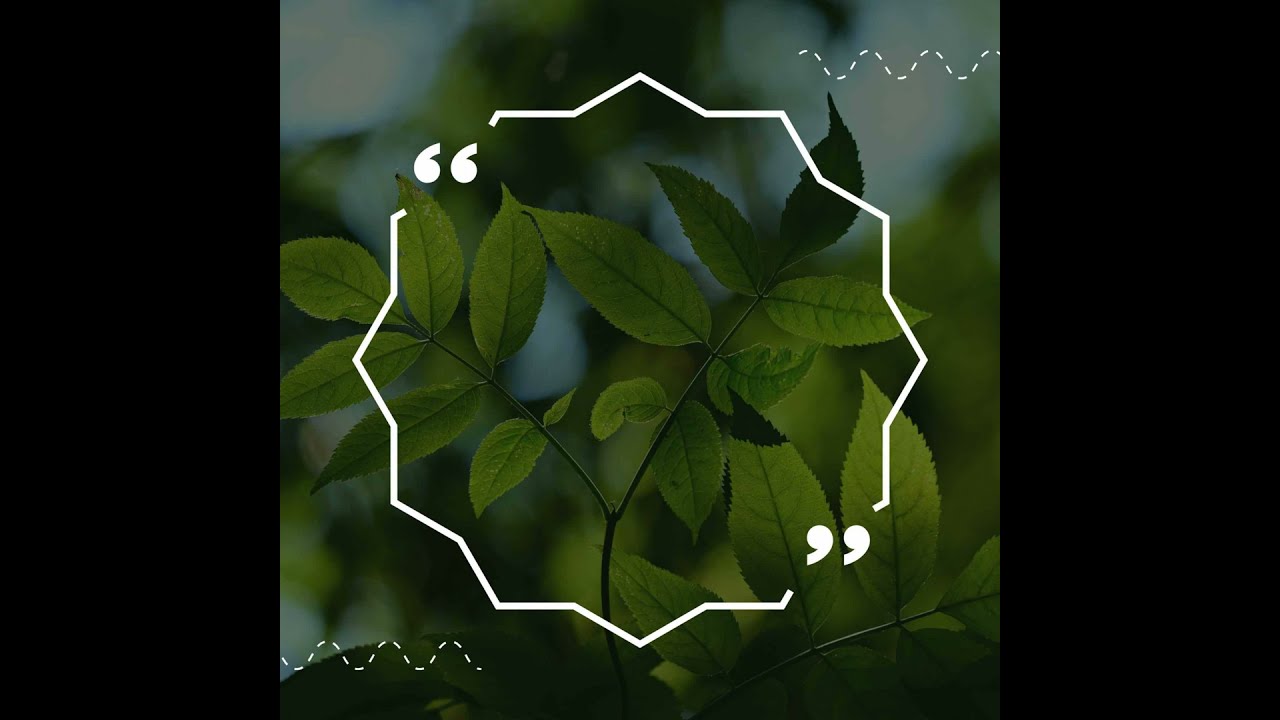The image depicts a close-up view of a small, young plant with vibrant green leaves and thin branches forming a Y shape, framed by a blurred, neutral green background that enhances the focus on the plant. The central part of the image showcases the plant's stems splitting into two main stalks, each adorned with pairs of sunlit leaves. Surrounding the plant is a jagged, multi-edged border, similar to a hexagon but with more sides, creating a dynamic, geometric overlay. Within this border, there are prominent bold quotation marks in the top left and right corners, making it a versatile template for adding text. Additionally, in the top right and bottom left corners of the image, thin white dashed sine wave patterns add decorative elements to the composition. This detailed, plant-themed template can be effectively used for presentations or graphic layouts.